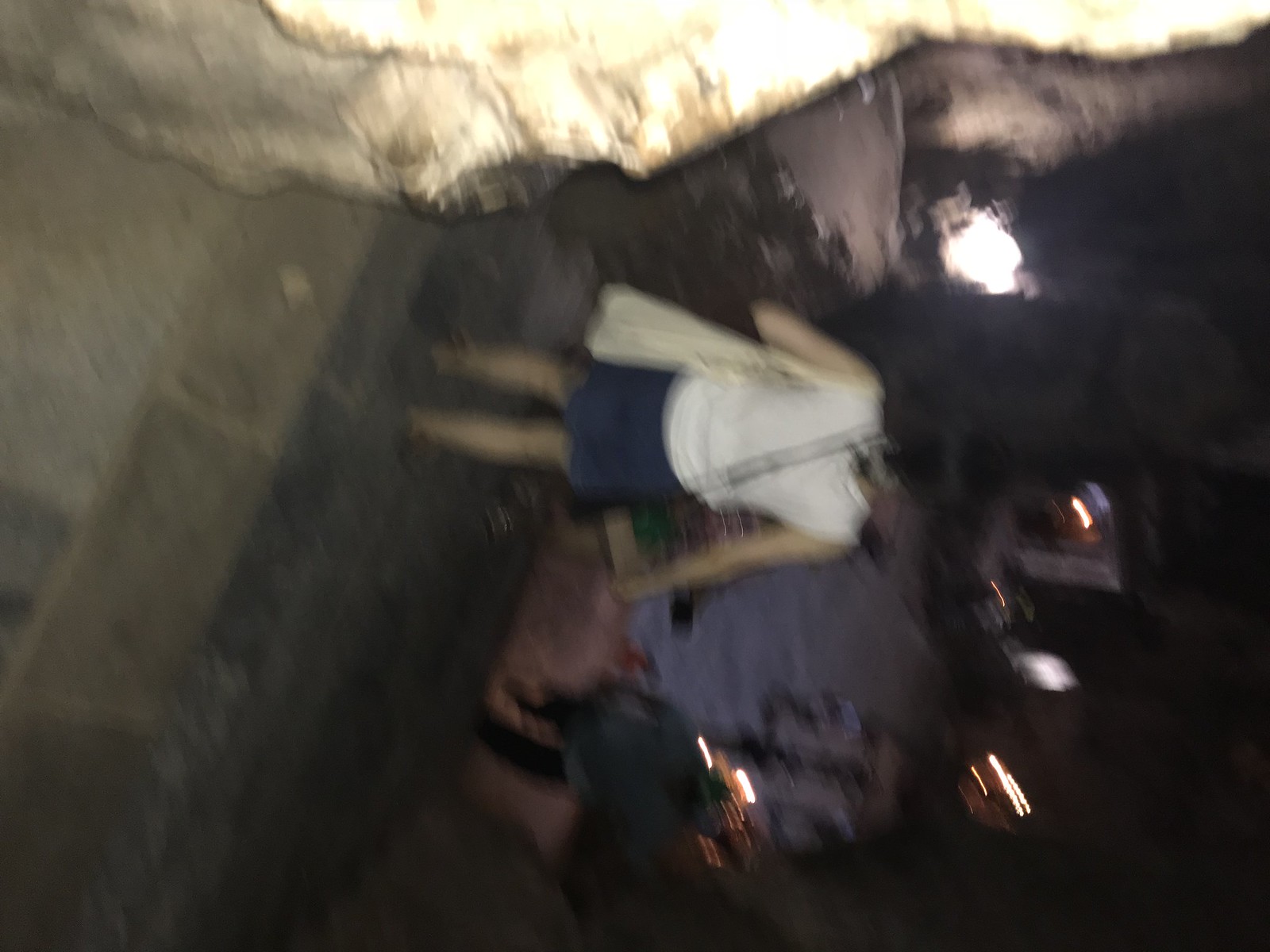This image, taken at night, is a very blurry and sideways photograph that seems to depict the back of a woman. The poor quality of the photo suggests that it was taken either with a very low-quality camera or with significant camera shake. The woman is wearing a white sleeveless top and a black, possibly knee-length skirt, which could also be interpreted as black shorts due to the blurriness. A line running diagonally across her back might be a handbag strap. The setting appears to be at an upward elevation, likely looking down from some stone steps, which are also blurred and indistinct. The floor she is standing on appears to be made of dark and light-colored slate stone. There is a light tan and white shape at the top of the photo, potentially the edge of a drape, and a round circle of light to the right. There are also some blurry, indistinct lights and a blob of light purple and pink in the background, making it difficult to discern the exact location or context of the scene. No text is visible in the image.